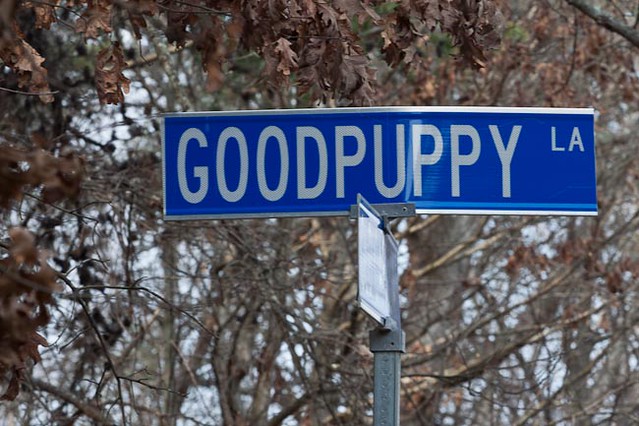The photograph captures a unique street sign situated outdoors, viewed against a backdrop of tall, partially barren trees, hinting at autumn or winter. The sign itself has a striking cobalt blue background with white text reading "Good Puppy," presented as a single word, and "L.A." in smaller letters at the top right, suggesting it could be located in Los Angeles or denote "Lane." The metal sign features a narrow stainless steel strip running along the left edge, top, and bottom, reflecting light off its polished surface. The blue sign is slightly damaged, with a noticeable bend between the 'U' and the 'P', creating a lighter, strained section in the metal. It is mounted on a standard gray steel pole at an intersection where another street sign is facing away, making it unreadable. The foliage surrounding the sign includes both green and numerous brown, dried leaves, indicating that the deciduous trees are either sick or out of season. The sky is clear, visible through the tree branches, adding to the serene yet somewhat desolate ambiance of the scene.